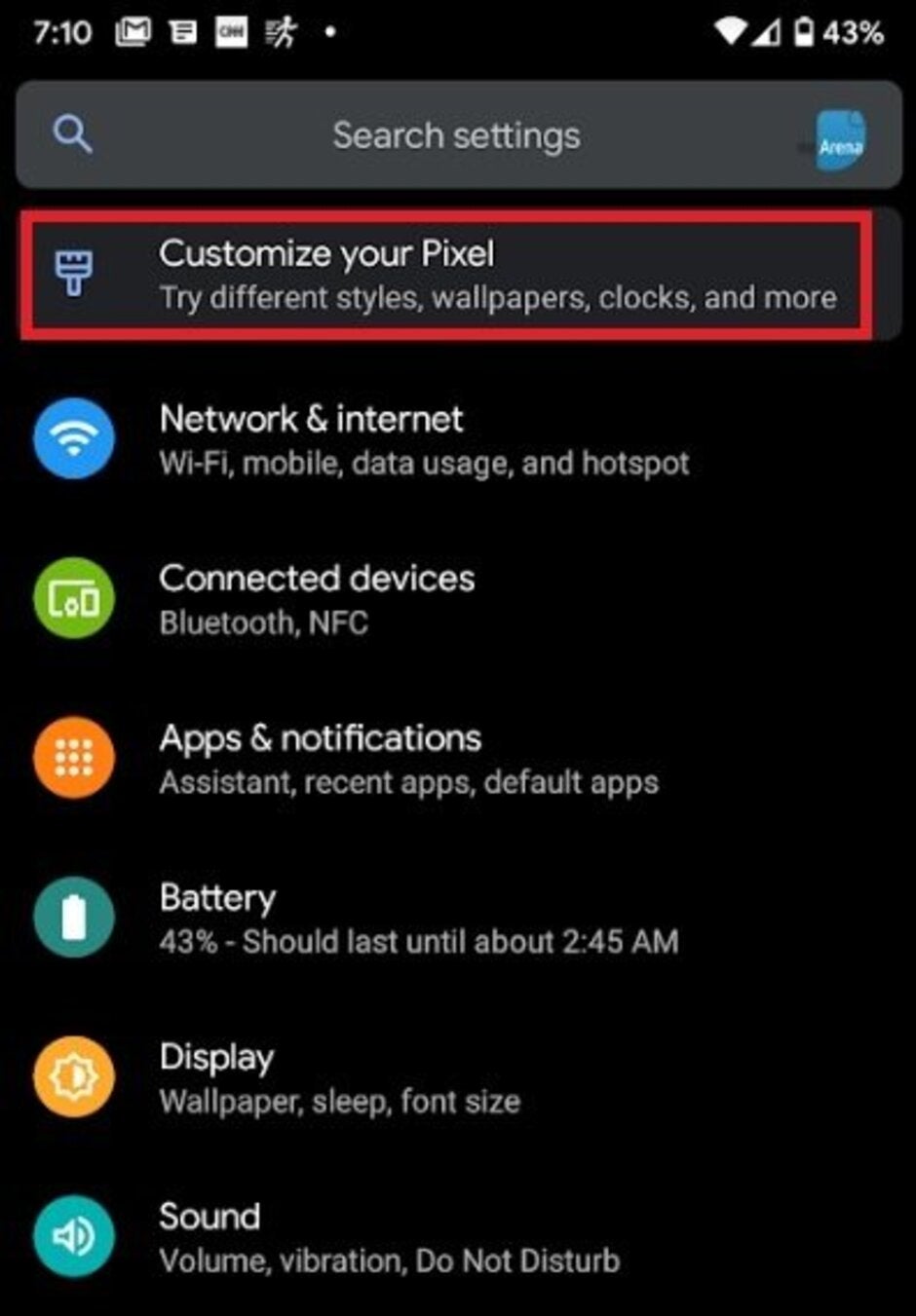This image is a screenshot from a smartphone with a black background. In the upper left-hand corner, the time is displayed as 7:10, though it's unclear whether it is AM or PM. Numerous small white icons are visible, including one depicting a male figure. On the upper right-hand corner, a battery icon shows a 43% charge. The wireless signal icon is half-filled, indicating mediocre signal strength, and there is a Wi-Fi icon as well.

Beneath these icons, a large gray rectangular search box is present, with the text "Search settings" written in very light gray font inside it. On the left side of this box, there is a search icon, which is a magnifying glass.

Against the black background, there is a list of settings items displayed in white font. At the top of the list, the item labeled "Customize your Pixel" is highlighted with a red outline. This item suggests trying different styles, wallpapers, colors, clocks, and more for the Google Pixel smartphone. 

Below it, the subsequent list items include:

1. "Network & internet" with a blue icon featuring the Wi-Fi signal symbol.
2. "Connected devices" marked with a green icon.
3. "Apps & notifications" accompanied by an orange circle icon containing nine small white dots arranged in a 3x3 grid.
4. "Battery" displaying the current charge at 43% and indicating the battery should last until approximately 2:45 AM.
5. "Display" without an icon.
6. "Sound" listed at the very bottom of the menu.